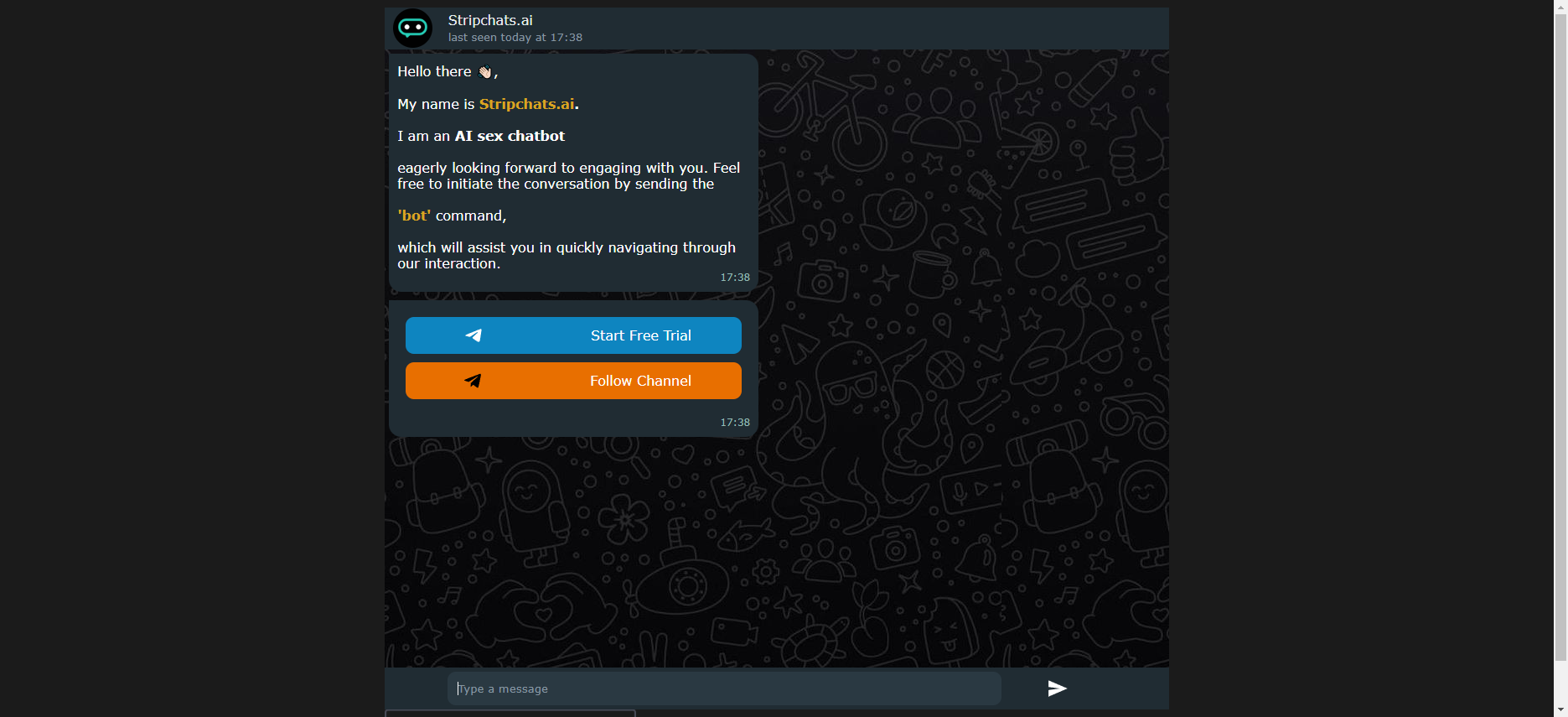The image depicts a digital interface with a predominantly black background, featuring a small square of information in the center. The focal point of the square appears to be the title "scriptchats.ai," noted alongside a use timestamp of "Friday at 1711" (military time). Within the square, the text initiates with a welcoming phrase: "Hello there," accompanied by a hand-wave emoji. It introduces, "My name is scriptchats.ai, I am an AI," followed by an indication that the AI assists with "chat" and "googling." The text encourages users to "initiate the conversation" but some words are obscured. Further instruction invites users to use "commands," highlighted in orange, to navigate through the platform efficiently. At the bottom of the square is a slender blue rectangle with the wording "Start Free Trial." Adjacent to it in orange, though partially unreadable, is a prompt beside a black arrow pointing upwards. Below the square is a text input field where users can enter messages, with an accompanying arrow pointing right.